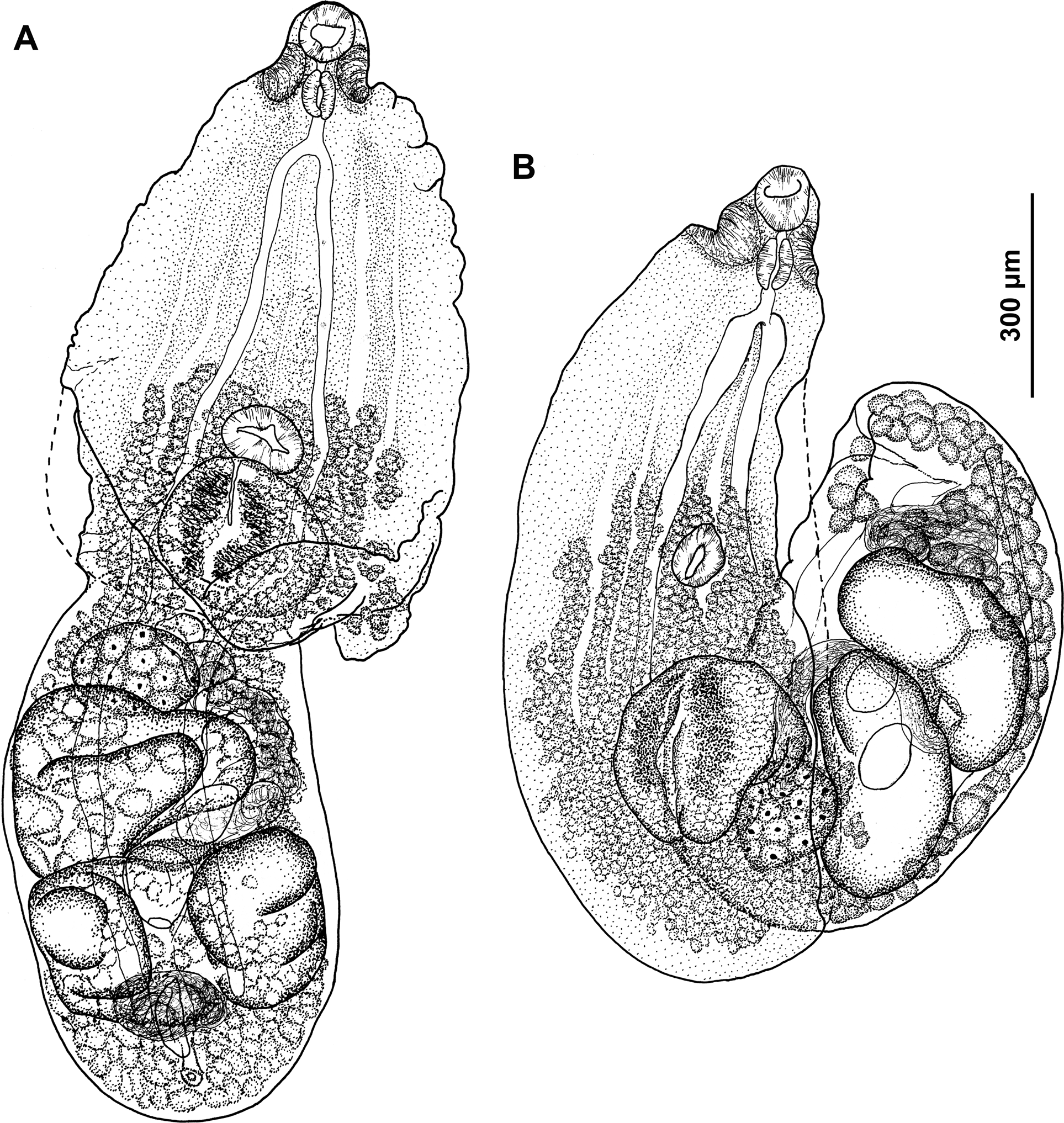This detailed black and white image depicts two intricate drawings, each labeled with 'A' on the left and 'B' on the right. Both drawings appear to represent the internal structures of small organisms or possibly anatomical diagrams. The drawing labeled 'A' shows a bulbous, oval shape that is broader at the bottom and tapering at the top. Near the top, there is a protrusion that curves up and then downward. A white line branches into two, leading into a darker gray area filled with various circular and oval shapes. Beneath this section, there is an elongated, oval structure with several internal compartments, densely packed with smaller shapes, giving the appearance of a sac hanging from the main body.

The drawing labeled 'B' shares some similarities with 'A' at the top. However, as it extends downward, it transforms into a more eggplant-like shape with analogous white protrusions leading into another grayish-black area. Below this area, instead of hanging down, the structure ascends and curves to the right, containing various shaped pockets. This drawing, more compact and rounded than 'A', seems to present a folded version of the organism depicted in 'A'. Running vertically on the right-hand side of the image is the notation "300 UM," indicating a scale or measurement line.